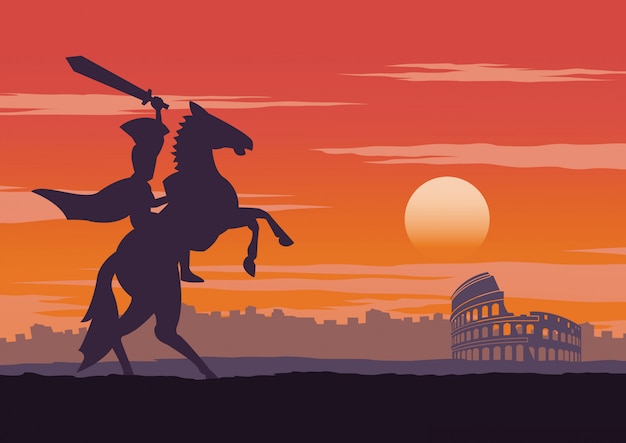In this rectangular illustration, a dynamic and dramatic scene unfolds. On the left side, a somewhat cartoon-like silhouette depicts a rearing horse standing on two legs, with a man astride its back. The man, dressed in clothing that evokes a bygone era, sports a flowing cape that billows dramatically in the wind, perhaps accentuated by the vigorous movement of the horse. Held aloft in his left hand, the man brandishes a long sword, adding a sense of impending action or heroism to the tableau.

The background is bathed in warm, golden hues, with the sun—a radiant orb—situated toward the lower right, casting an ethereal glow over the scene. The sun’s rays illuminate the remnants of an ancient-looking structure, reminiscent of Greek ruins or a Colosseum, its crumbling arches and columns partially visible. This historic ruin stands as a poignant reminder of a once-majestic edifice, now reduced to faded glory.

On the horizon, a faint line of buildings is sketched in brown, their detailed outlines hinting at a distant, perhaps long-forgotten civilization. The entire image, rendered in a cartoon style, blends the grandeur of historical elements with a whimsical artistic touch, creating a visually captivating narrative.